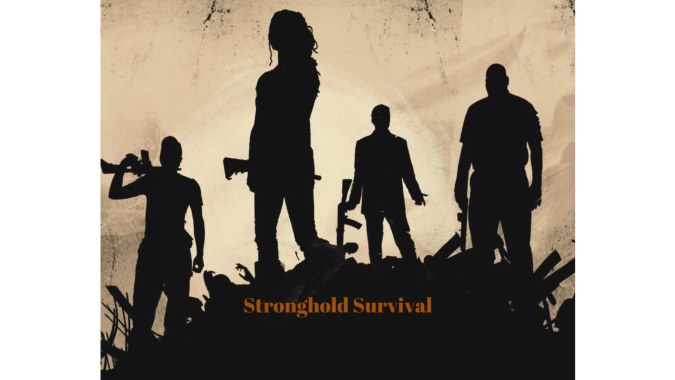The image appears to be a computer graphic poster titled "Stronghold Survival" set against a light brown to tannish background. Foregrounded against this backdrop is a dynamic scene of four silhouetted figures, three males and one female, rendered in dark black or brown shadows due to a light source positioned behind them. These figures stand atop a mound, which seems to consist of bodies or debris, with discernible remnants like a hand sticking out. Starting from the left, the first figure is a male with his right elbow bent, holding a gun over his shoulder. The second figure, likely a female indicated by long hair, holds a weapon—possibly an axe—at her waist. Positioned higher and to her right, the third male faces away, gripping a gun aimed to the left side of his body. The fourth figure mirrors this stance, also holding a gun down at the left side of his body. The combination of silhouetted figures and their strategic poses evokes a narrative of survival and resilience amidst chaos.